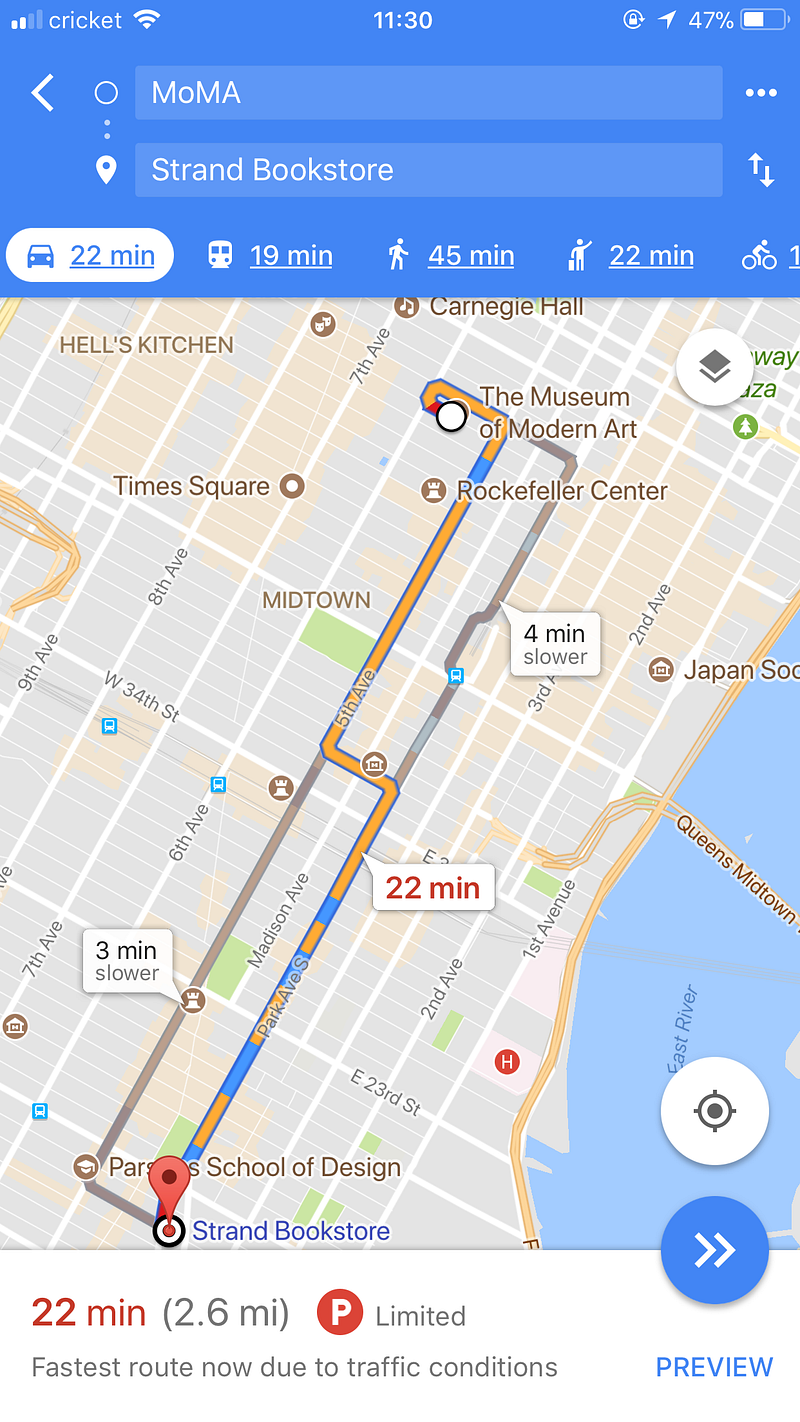This image is a screenshot of a Google Maps directions result displayed on a smartphone. At the very top, within a blue background banner, we see various icons: a cellular reception icon showing two out of five bars, the word "Cricket," and a Wi-Fi symbol. Centrally positioned at the top, the time is displayed as 11:30, while the upper right corner includes several additional icons along with a battery indicator showing 47% charge.

Below this banner, the primary section with a white background features search details and a map. The search details specify "MoMA" as the starting point and "Strand Bookstore" as the destination. The map prominently displays a detailed view of Midtown Manhattan, highlighting the route between these two locations with driving directions.

Above the map, various transportation options are listed with their corresponding travel times: driving (22 minutes), public transportation (19 minutes), walking (45 minutes), and ride share or taxi (22 minutes).

At the bottom of the image, further route details are provided: "22 minutes, 2.6 miles," with a note indicating limited parking availability. It also remarks that this is the fastest route at the moment due to current traffic conditions.